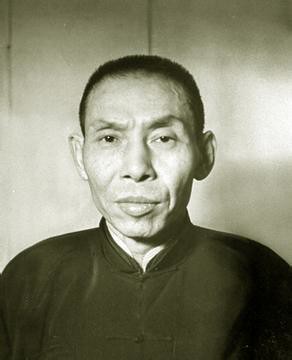The black-and-white photograph features an older Asian gentleman, approximately in his mid-40s, standing in front of a plain, paneled wall made from wooden planks. The man is dressed in a traditional Chinese top, identifiable by its ornate collar and central buttons. His dark garment with a stand-up collar accentuates his serious and focused expression, as he stares directly at the camera. The portrait, captured from his head to mid-chest in a photographic style of realism, reveals his short black hair, slightly wrinkled forehead near the temples, and large ears. The lighting illuminates him, casting a natural glow from the top right of the image, enhancing the textures and details of both his face and the background.